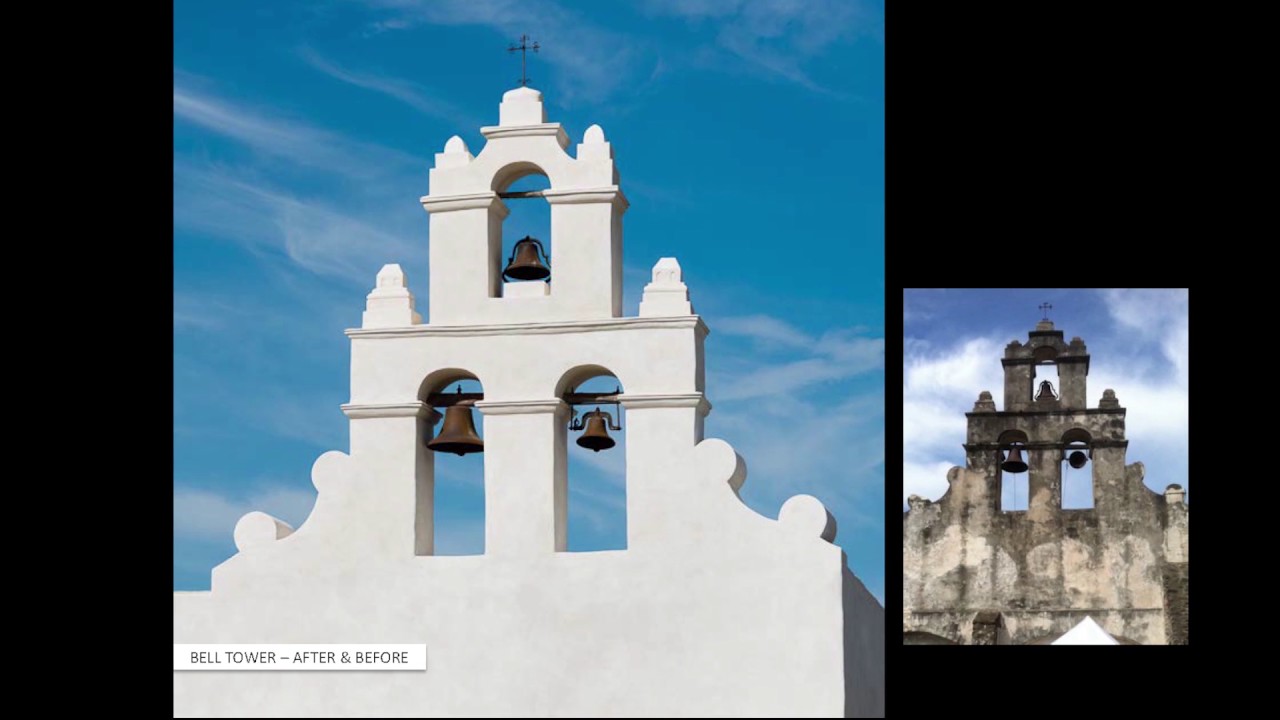The image consists of two side-by-side photographs of a bell tower, possibly reminiscent of the Alamo or a church tower. Both photos are set against a clear blue sky. The left photograph, labeled "after," showcases a recently restored bell tower that is bright white, smooth, and clean with three brown bells near the top. In contrast, the right photograph, labeled "before," depicts the same bell tower in a visibly deteriorated state, looking dirty, grey, and discolored, with its aged surface displaying signs of wear and a lack of detail. This juxtaposition highlights the significant restoration efforts undertaken to rejuvenate the historic structure.